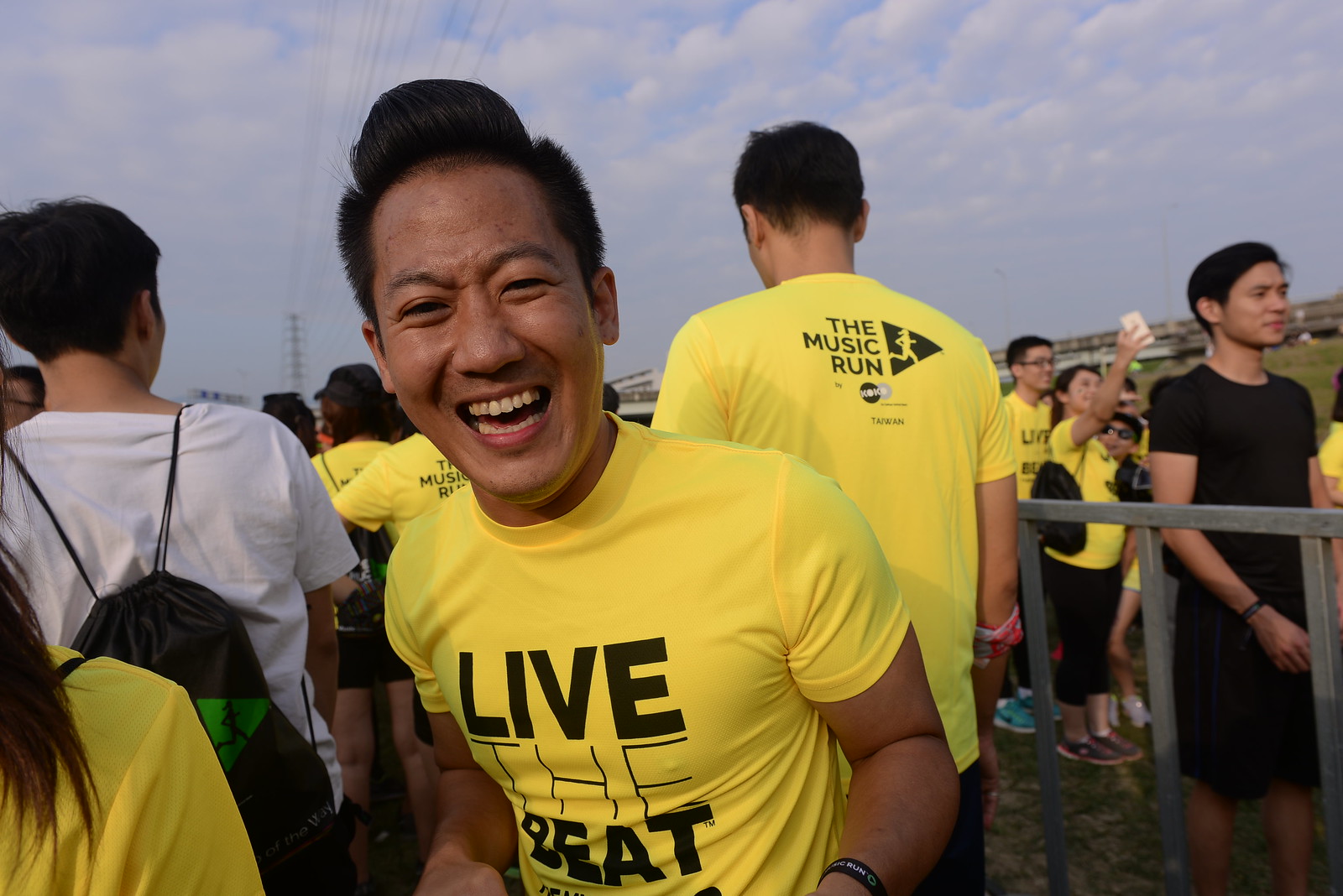In this vibrant, full-color outdoor photograph, a young Asian man is prominently featured, beaming joyfully as he turns to face the camera. He is dressed in a bright yellow t-shirt emblazoned with the slogan "Live the Beat," reflecting a lively atmosphere. Behind him, another person wearing the same yellow shirt displays the back which reads "The Music Run," accompanied by a black triangle containing the image of a woman running. This underscores it being part of a well-attended event, likely focused on music and running. The scene shows a clear, sunny day with patches of clouds scattered above an expansive grass field. Surrounding the smiling young man, people mostly face away, hinting at a line formation he's momentarily turned away from to capture this cheerful snapshot. On the right, another woman dressed similarly is engaged in taking a selfie, enhancing the sense of communal enjoyment and festivity. Iron bars in the background further emphasize the orderly nature of the gathering.